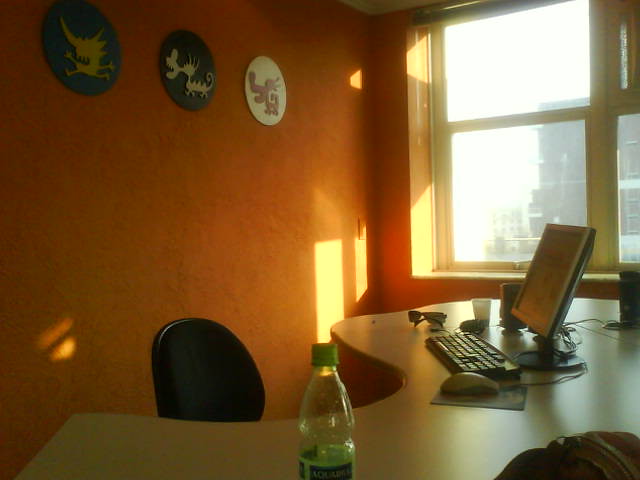This detailed photo captures an interior office scene featuring a large, curvy white desk that almost resembles a table. Positioned in front of the desk is a black chair. On the desk, various objects are meticulously arranged: a black computer monitor, a white mouse on a mouse pad, a pair of sunglasses, a cup, and a few other miscellaneous items. Notably, a bottle of water stands upright in the foreground. The room's walls are painted a vibrant orange and adorned with three circular artistic frames, each showcasing abstract designs with creatures at their center. These frames depict what appear to be dragons and dogs, adding a touch of whimsy and creativity to the space. A window in the background reveals a high-rise view with other buildings visible in the distance, enhancing the office's sense of openness and connectivity to the urban environment outside.